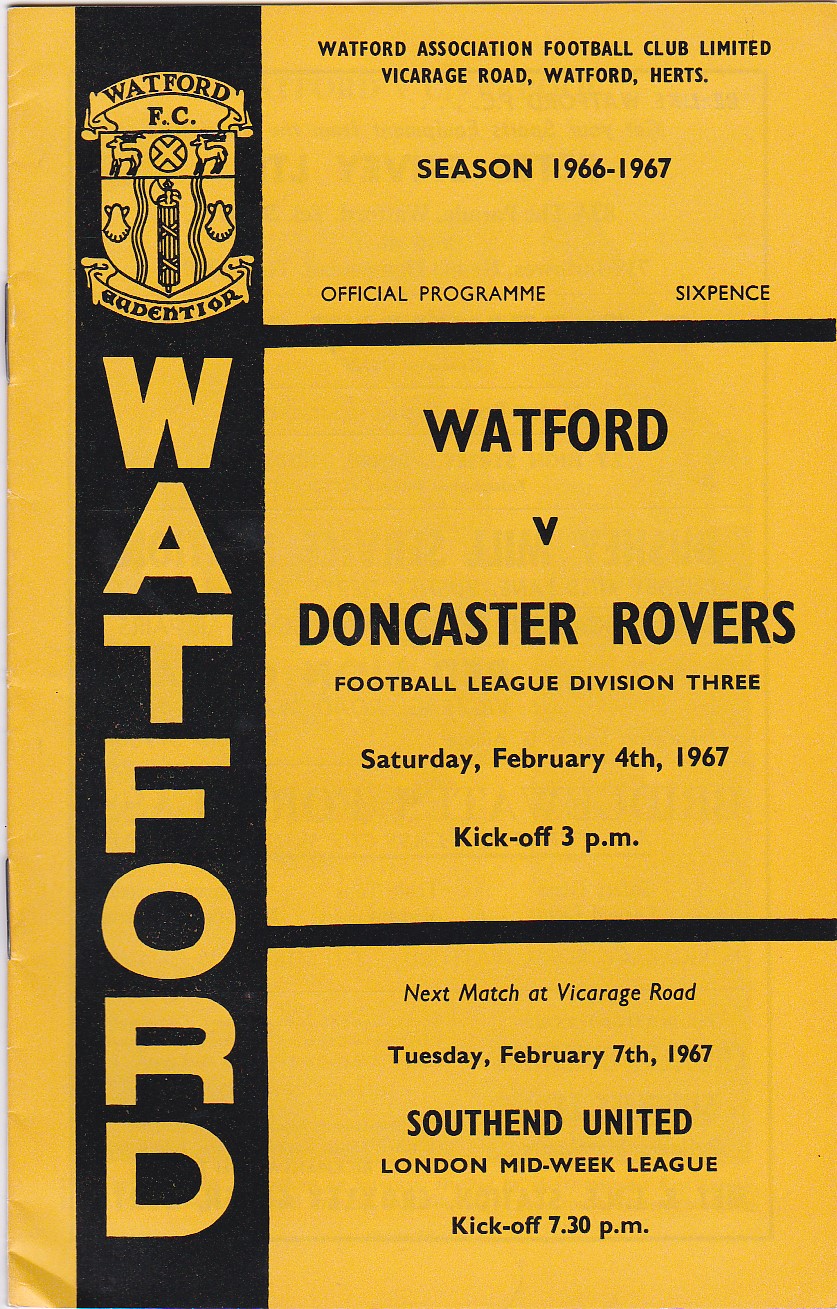The image depicts the front cover of a football program for the Watford Association Football Club. The cover features an orange background with black text. The top of the program includes the official header: "Watford Association Football Club Limited, Vicarage Road, Watford Herts, Season 1966-1967, Official Program, Sixpence." The main event advertised is the match between Watford and Doncaster Rovers in the Football League Division III, scheduled for Saturday, February 4, 1967, with kickoff at 3pm. Additionally, the cover mentions the next home game against Southend United in the London Midweek League on Tuesday, February 7, 1967, with kickoff at 7:30pm. On the left side of the program, a white vertical band features the Watford FC logo at the top, comprising a shield with a circle containing an X, flanked by two goats. Below the logo, the name "Watford" is prominently displayed.